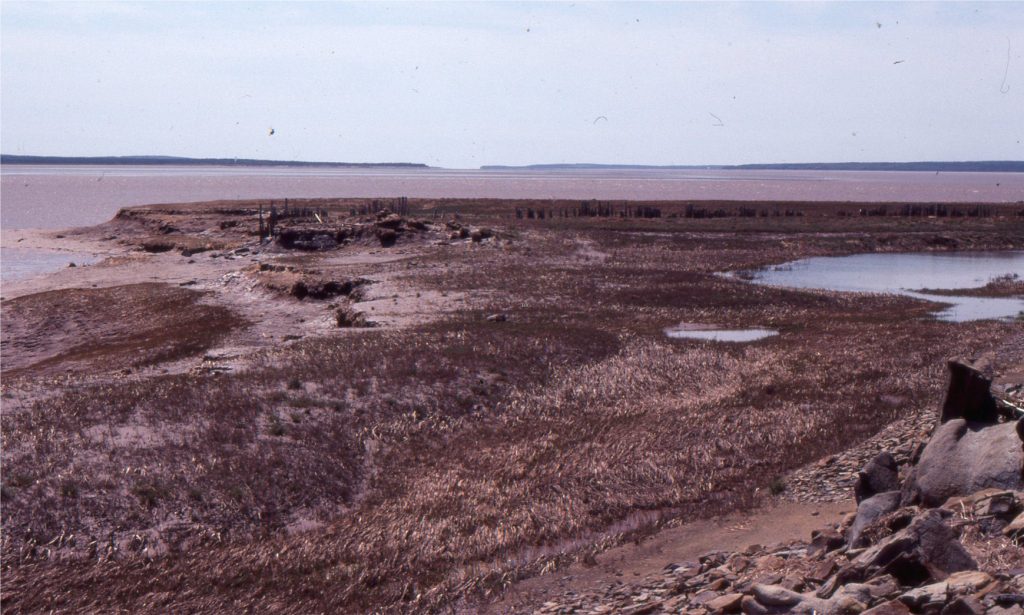This is a photograph of a barren landscape taken on a gray, cloudy day. The sky dominates the top fourth of the image with its light blue, slightly grayish hue, creating an overcast atmosphere. The horizon reveals a strip of distant land, with very gray water lying just beyond it. 

In the foreground, notably on the right side, the land is darker brown and speckled with larger rocks and stones of varying shapes and sizes. These rocks are rough in texture and come in different shades of brown. A small pond or body of water is also present on the right, nestled within the landlocked area. To the left, more brown rocks fade into another body of gray water, giving an impression of multiple small lakes or ponds scattered throughout the scene.

Sparse, brown vegetation dots the landscape, with some tiny vertical brown structures visible in the distance, blending seamlessly with the natural surroundings. The overall color palette is muted, consisting mainly of earthy tones, grays, and browns, contributing to the desolate feel of the terrain.